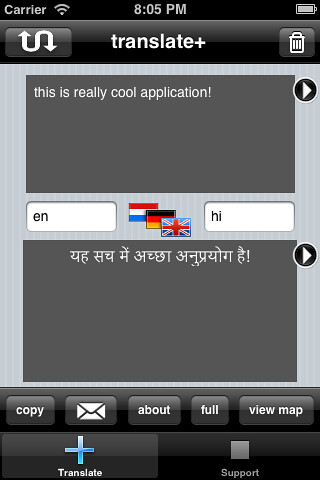This vertically aligned, smaller-sized rectangular image appears to be a screenshot from a cell phone taken at night, as indicated by the time 8:05 PM displayed in white numbers at the top center. The phone shows a fully charged battery icon on the far right and full Wi-Fi signal bars on the left, along with the word "carrier" in gray on a black background.

Below this top bar, the screen features an app called "Translate Plus." A white heading with the app's name is prominently displayed, flanked by a recycle bin icon on the right and a curved up-and-down arrow icon on the left. The primary screen area is divided into several sections, starting with a dark gray rectangular area with the text "This is a really cool application!" written in gray and possibly highlighted to catch the viewer's attention.

Centrally, the image showcases three overlapping flags: the Union Jack of the United Kingdom, the flag of Luxembourg, and the flag of Germany. Directly beneath these flags are two small white rectangular boxes labeled "EN" for English and "HI" for Hindi, indicating the language translation options the app supports.

A second dark gray rectangular section appears further down, displaying a series of white symbols ending with an exclamation mark, reflecting a user-friendly interface. Finally, at the bottom of the screenshot, there are several dark gray buttons with white text: "Copy," an email envelope icon, "About," "Full," and "View Map," offering additional functionalities within the app.

Overall, the screenshot effectively showcases the features and user interface of the "Translate Plus" app, emphasizing its practicality and accessible design.